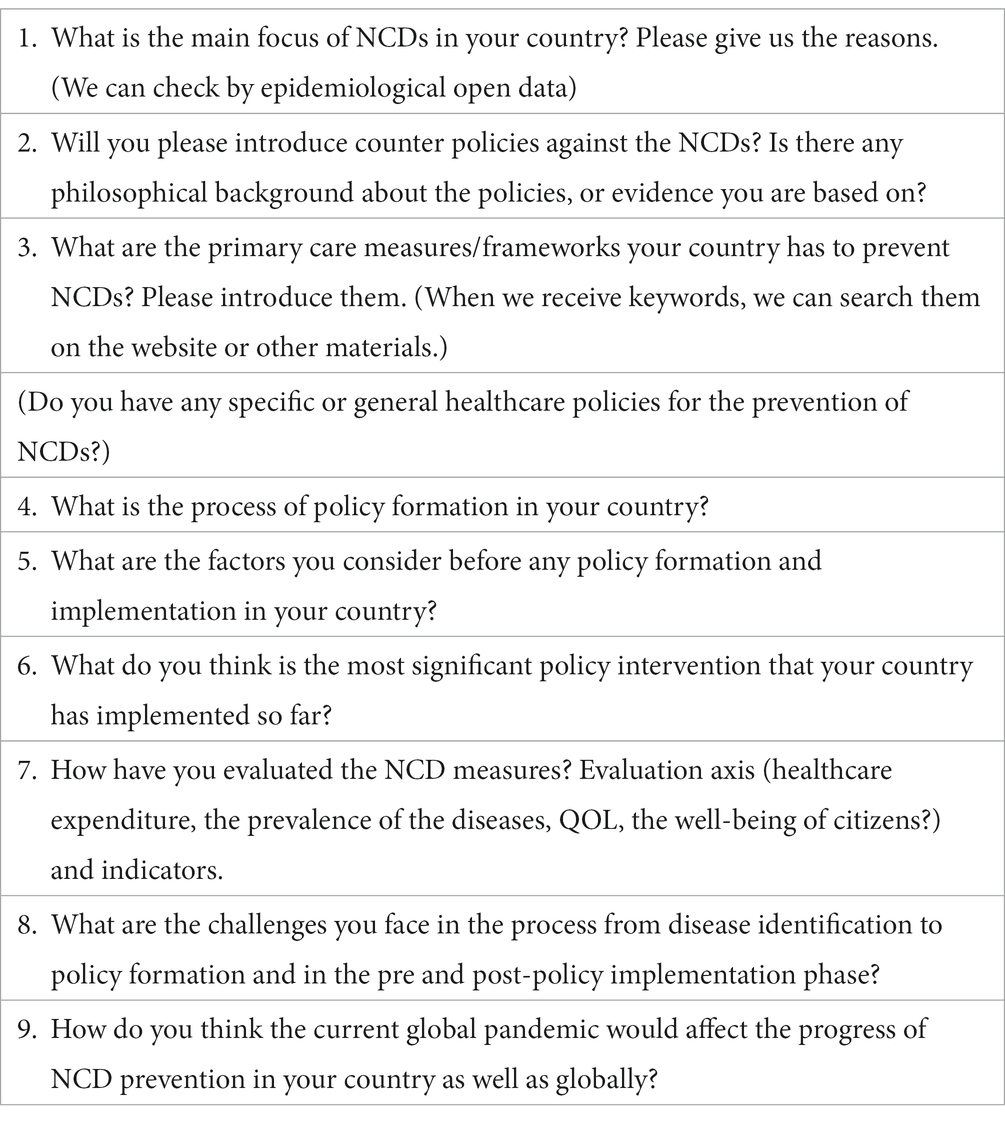A vertical list of nine questions, concerning non-communicable diseases (NCDs), is displayed against a white background. Each question is enclosed within its own rectangular box, separated by gray lines for clarity. The entire image is framed with a light gray border. The questions, written in black text, are numbered sequentially:

1. "What is the main focus of NCDs in your country? Please give us the reasons. (We can check by epidemiological open data)."
2. "Will you please introduce counter policies against the NCDs? Is there any philosophical background about the policies or evidence you are based on?"
3. "What are the primary causes/frameworks your country has to prevent NCDs? Please introduce them. (When we receive keywords, we can search them on the website or other materials)."
   - (Follow-up: "Do you have any specific or general health care policies for the prevention of NCDs?")
4. "What is the process of policy formation in your country?"
5. "How is the effectiveness of these policies evaluated?"
6. "What challenges do you face in implementing these policies?"
7. "What role do various stakeholders (government, private sector, civil society) play in addressing NCDs?"
8. "Are there any ongoing or planned public awareness campaigns regarding NCDs?"
9. "How does your country collaborate with international organizations on NCD issues?"

This structured and detailed inquiry aims to comprehensively understand the approaches and challenges related to managing NCDs across different nations.